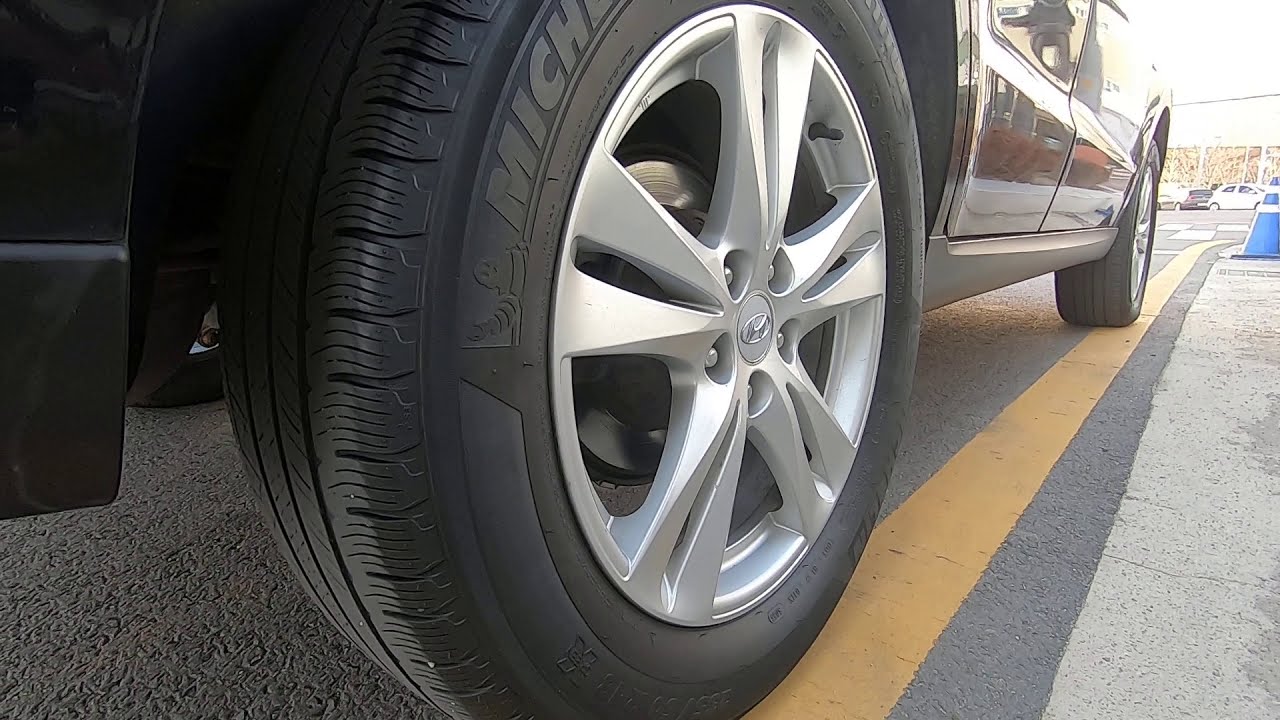The image depicts a close-up of a car wheel, likely the front left one, as evidenced by the reflection of the side mirrors on the door nearby. The car appears to be either brand new or meticulously cleaned, characterized by gleaming body panels and spotless black tires. The silver metallic rim, likely chrome or highly polished, features ten split spokes with five lug nuts, and displays part of the Michelin logo, indicating Michelin brand tires with new treads. The tire is situated on a yellow line on an asphalt parking lot. This lot also features an orange stripe running along the right side of the car, with the wheels overlapping it slightly. In the background, there is a blue cone in the corner of the parking space and a number of parked cars visible in the distance. Additionally, reflections on the car's tan-ish colored body show the side mirrors and a red truck, further indicating its reflective and clean surface.